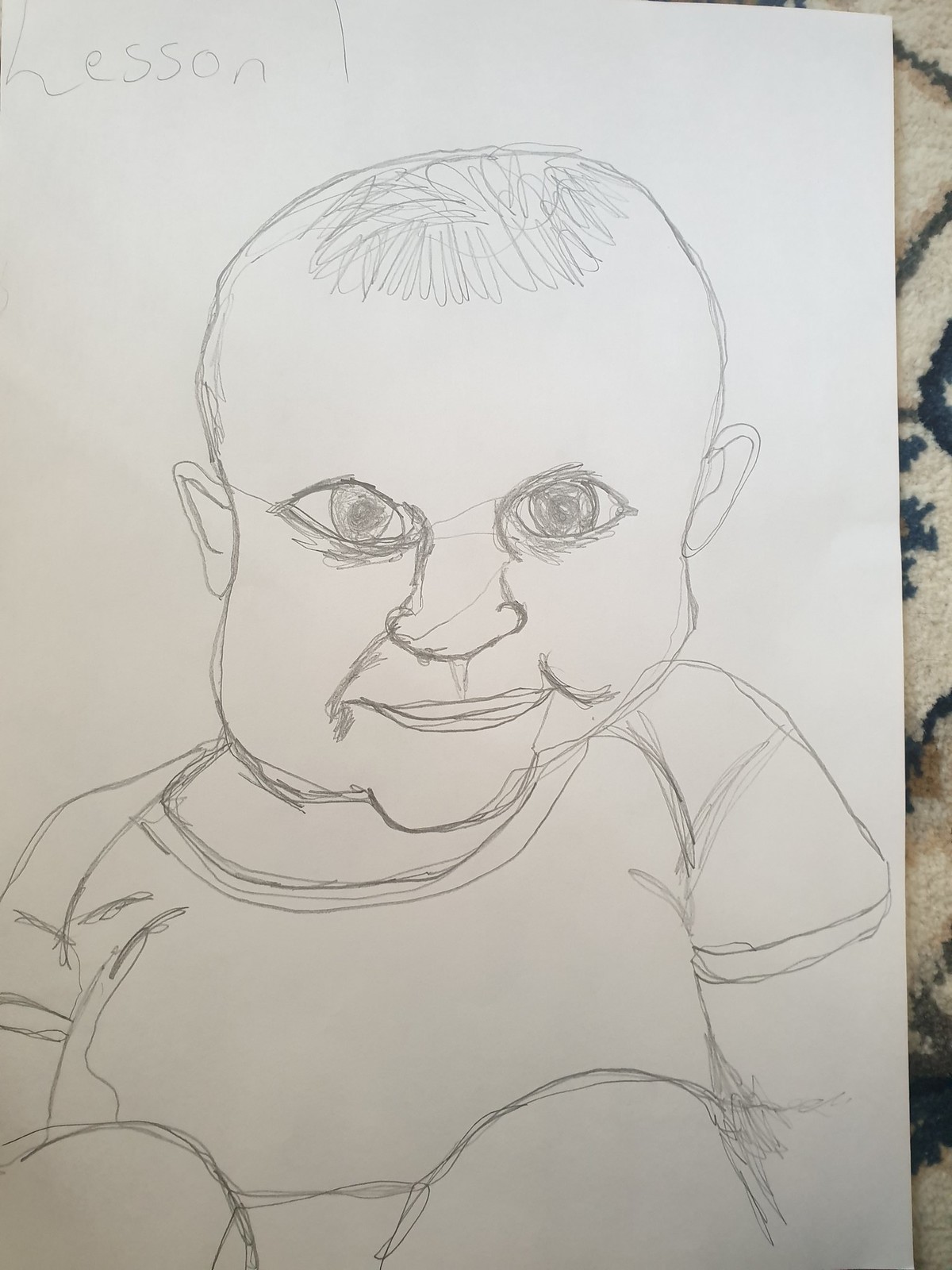This is a pencil and paper drawing of a slightly out-of-proportion baby wearing a fold-over shoulder t-shirt. The baby’s head is misshapen, with uneven, wonky ears and extremely large eyes. The nose and mouth are also depicted, contributing to the simple, amateur style of the drawing. The neck is not visible, but the little chest is noticeable below the t-shirt. The baby appears chunky with characteristic baby fat. The body posture is ambiguous, with limbs either pulled up towards the chest or drawn disproportionately, curving in front of the torso.